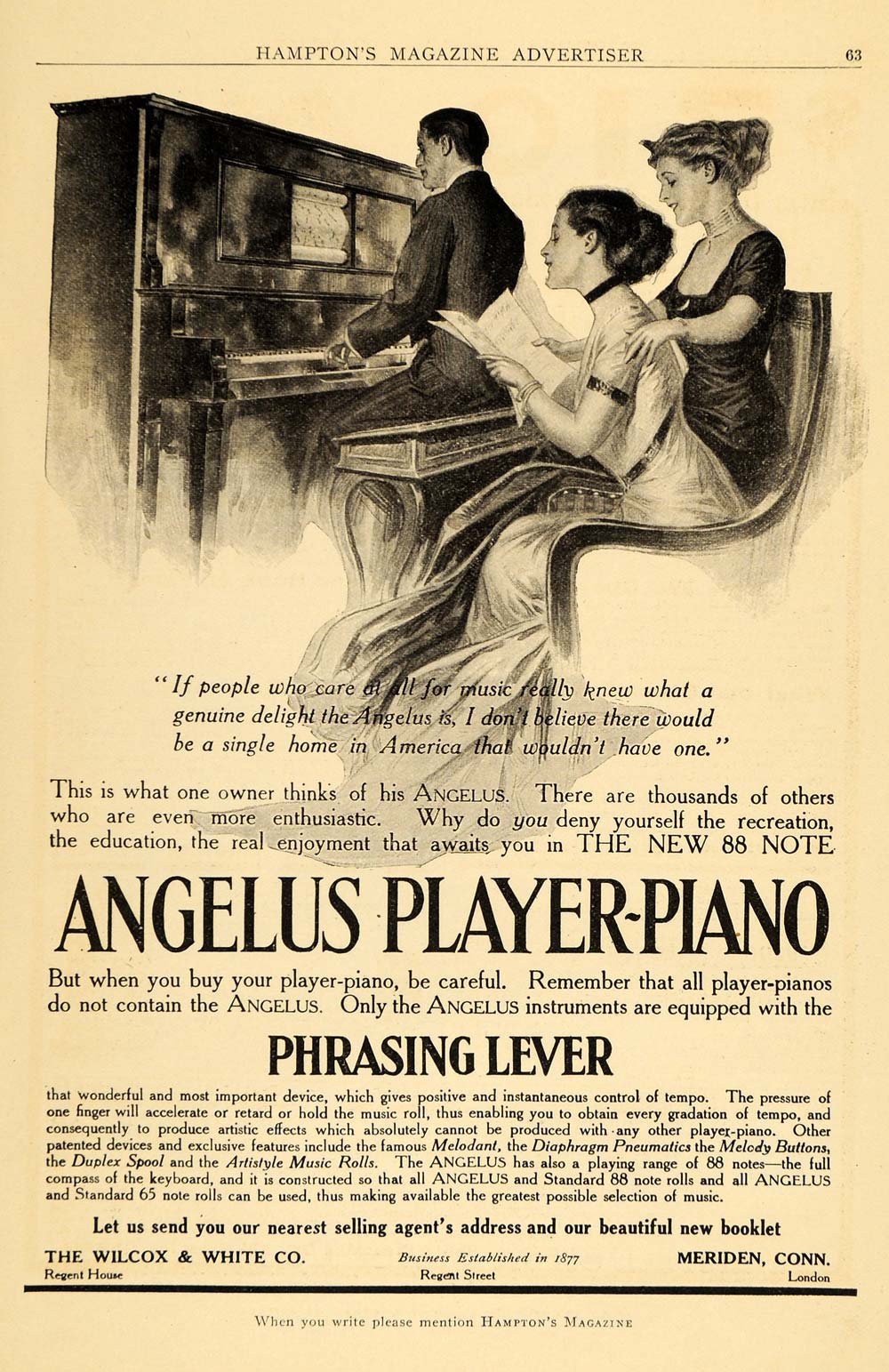This vintage advertisement from Hampton's Magazine, page 63, promotes the Angelus Player Piano. Set against a yellowed background tinged by age, the central illustration features a man playing a player piano. Though the piano can play itself, the man engages directly with it, adding a personal touch. To his right, two women share a chair; one has her hands on the other’s shoulders, accentuating her unusually short arms. Both women are in long dresses, possibly singing or reading music as they participate in the musical moment.

The caption under the illustration captures an enthusiastic testimonial: "If people who care at all for music really knew what a genuine delight the Angelus is, I don't believe there would be a single home in America that wouldn't have one. This is what one owner thinks of his Angelus. There are thousands of others who are even more enthusiastic. Why do you deny yourself the recreation, the education, the real enjoyment that awaits you in the new 88 note?" Boldly, the advertisement declares, "ANGELUS PLAYER PIANO."

Buyers are cautioned to ensure their player piano is a genuine Angelus, emphasizing that "only the Angelus instruments are equipped with the phrasing lever." Further text offers to send potential customers the address of the nearest selling agent and a beautiful new booklet, with the ad concluding by noting "The Wilcox and White Co., Regent House, business established in 1877, Regent Street, Meriden, Connecticut, London." At the bottom, it advises readers, "When you write, please mention Hampton's Magazine."